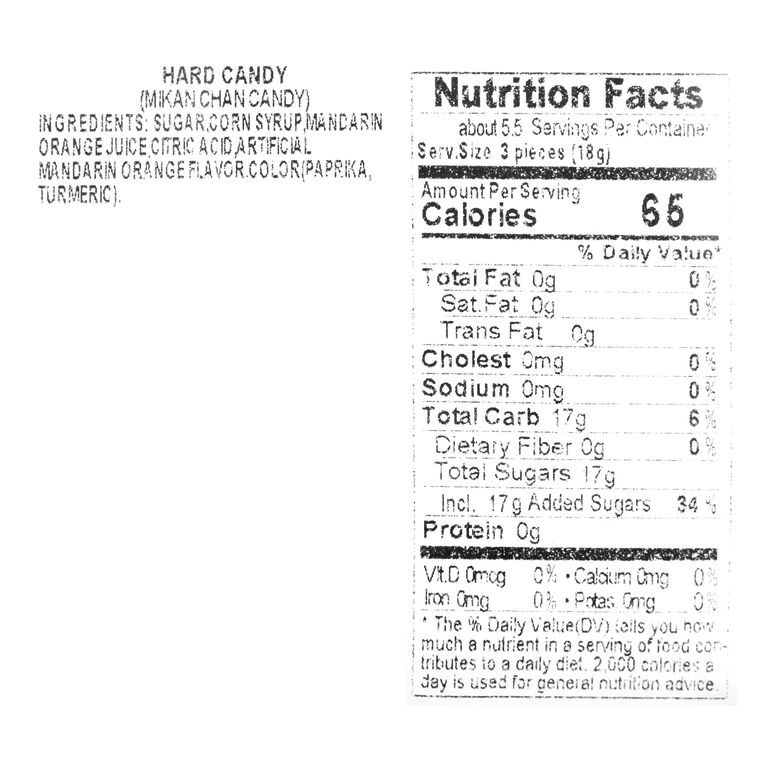The image is a detailed close-up of the nutritional facts and ingredient list on the back of a hard candy package. On the left, the text prominently displays "Hard Candy" and in parentheses "Mikan Chan Candy." The ingredients listed are: sugar, corn syrup, mandarin orange juice, citric acid, artificial mandarin orange flavor, with colorants paprika and turmeric. On the right side, the standard rectangular nutrition facts label indicates there are about 5.5 servings per container. Each serving size is three pieces or approximately 8 grams. The nutritional breakdown per serving includes: 65 calories, 0 grams of total fat, 0 grams of saturated fat, 0 grams of trans fat, 0 milligrams of cholesterol, 0 milligrams of sodium, 17 grams of total carbohydrates, 0 grams of dietary fiber, 17 grams of total sugars including 17 grams of added sugars, and 0 grams of protein. The label also notes that there are 0% daily values for Vitamin D, calcium, iron, and potassium. The provided percent daily value information helps consumers understand the contribution of these nutrients within the context of a 2,000-calorie daily diet.